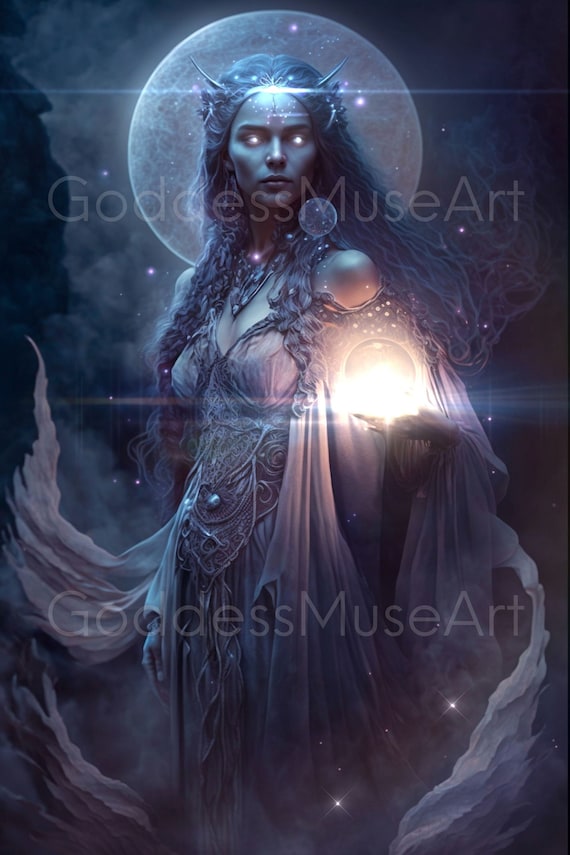This digital artwork titled "Goddess Muse Art," featuring intricate watermarks at the top and bottom middle, depicts a captivating, ethereal woman set against a dark, star-speckled night sky. She is adorned with elongated, elven ears and a radiant tiara, exuding a celestial aura. Encircling her head is a luminous moon-like halo. Her eyes, piercing and bright white, emit a glowing light. She wears a flowing, ornate dress in hues of bluish-purple and lilac, embellished with drapes and a boned corset. The garment seems to billow organically, as if animated by a gentle breeze, with tendrils that extend gracefully to the sides. Clutched in her left hand is a glowing white orb—the only element breaking the monochromatic palette besides her eyes. Her long, flowing hair, fluttering elegantly, adds to her otherworldly appearance. The ambiance is further accentuated by a subtle glow emanating from her shoulder, enhancing the mystical and galactic feel of this intricately detailed image.